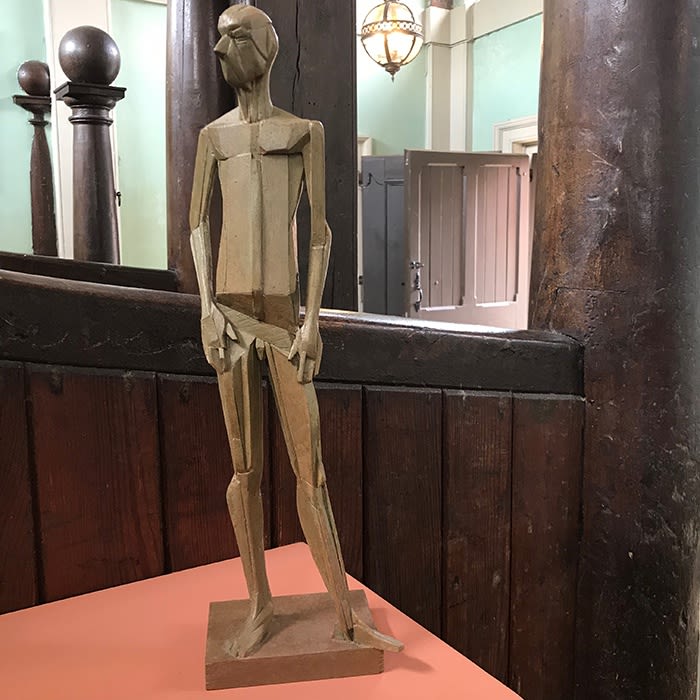This color photograph captures a modern, artistic wooden sculpture of a human figure as its focal point. The statue, primarily brown with varying shades, is portrayed in a slightly turned profile, facing the viewer with its head angled to the right. The human figure is characterized by planed shapes, such as rectangles and triangles, and stands on a short, wide square base placed atop a reddish-hued, square table. The figure exhibits detailed features like eyes, nose, faint hair, and hands that rest on its legs. It lacks a mouth and clothing, conveying a minimalist aesthetic.

The background sets the sculpture in what appears to be a museum-like environment, featuring a dark brown wooden half wall crowned with a column on the right side. Behind the sculpture are mint green walls complemented by white trim along the ceiling and pillars descending into the corners. Several wooden doors and additional wooden pillars are present, inferring a sophisticated interior with elements of realism, possibly indicating this piece as contemporary work by the artist Bridget Harris.